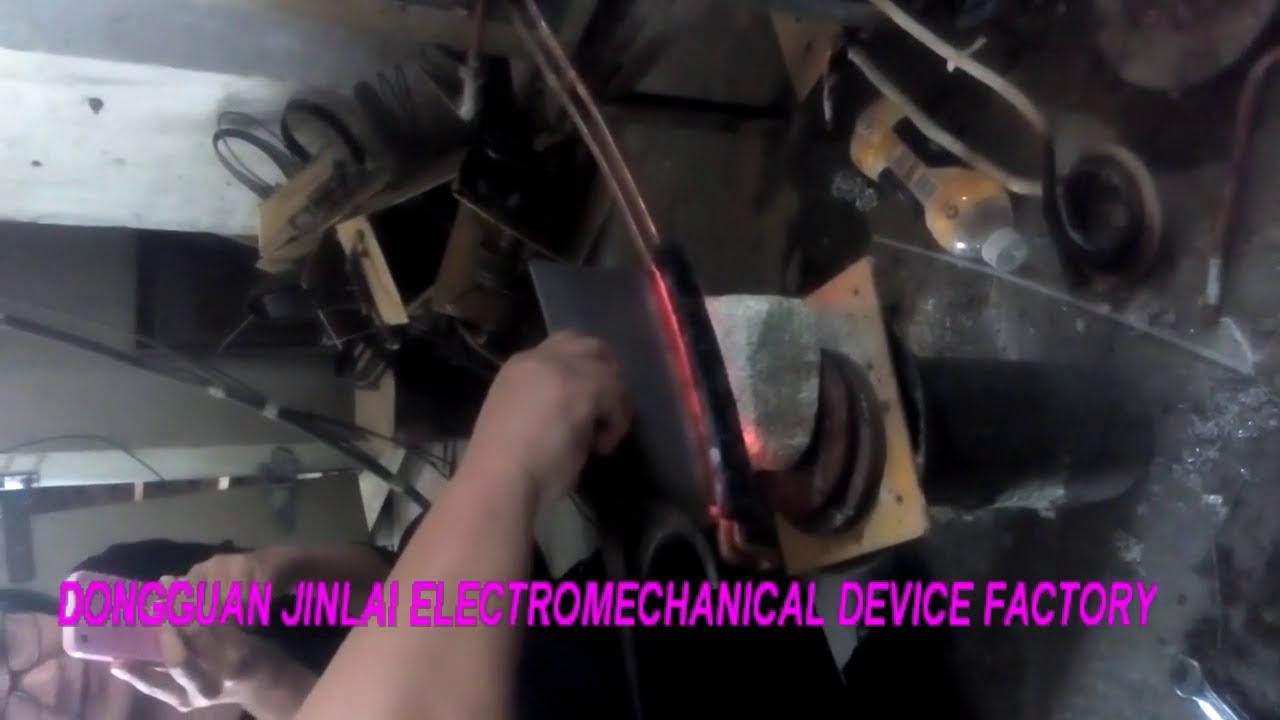In this detailed image from the Dongguan Jinlai Electromechanical Device Factory, the scene features various elements of a metalworking shop. Dominating the center is a hand and forearm engaged in a precise task, holding a metal object that is being shaped or heated against another metal piece, evoking the image of a modern blacksmith. The arm appears to be manipulating the metal near electrified copper cables, with a gray granite-like stone forming part of the work surface. Scattered on the floor are various tools, including tongs and a hammer, and other apparatus essential for metalworking. A possibly repurposed stovepipe, welded to the floor, acts as a support structure. The floor itself is cluttered with broken glass and a discarded plastic drink bottle, adding to the industrial atmosphere. The overall image orientation suggests the picture was taken from a unique angle, requiring viewers to tilt their heads for proper perspective. Adding a human element, the background reveals an Asian woman holding a pink cell phone, capturing the ongoing work. Encapsulating the essence of this industrious environment, the bottom of the image prominently displays the text "Dongguan Jinlai Electromechanical Device Factory" in vivid pink capital letters.